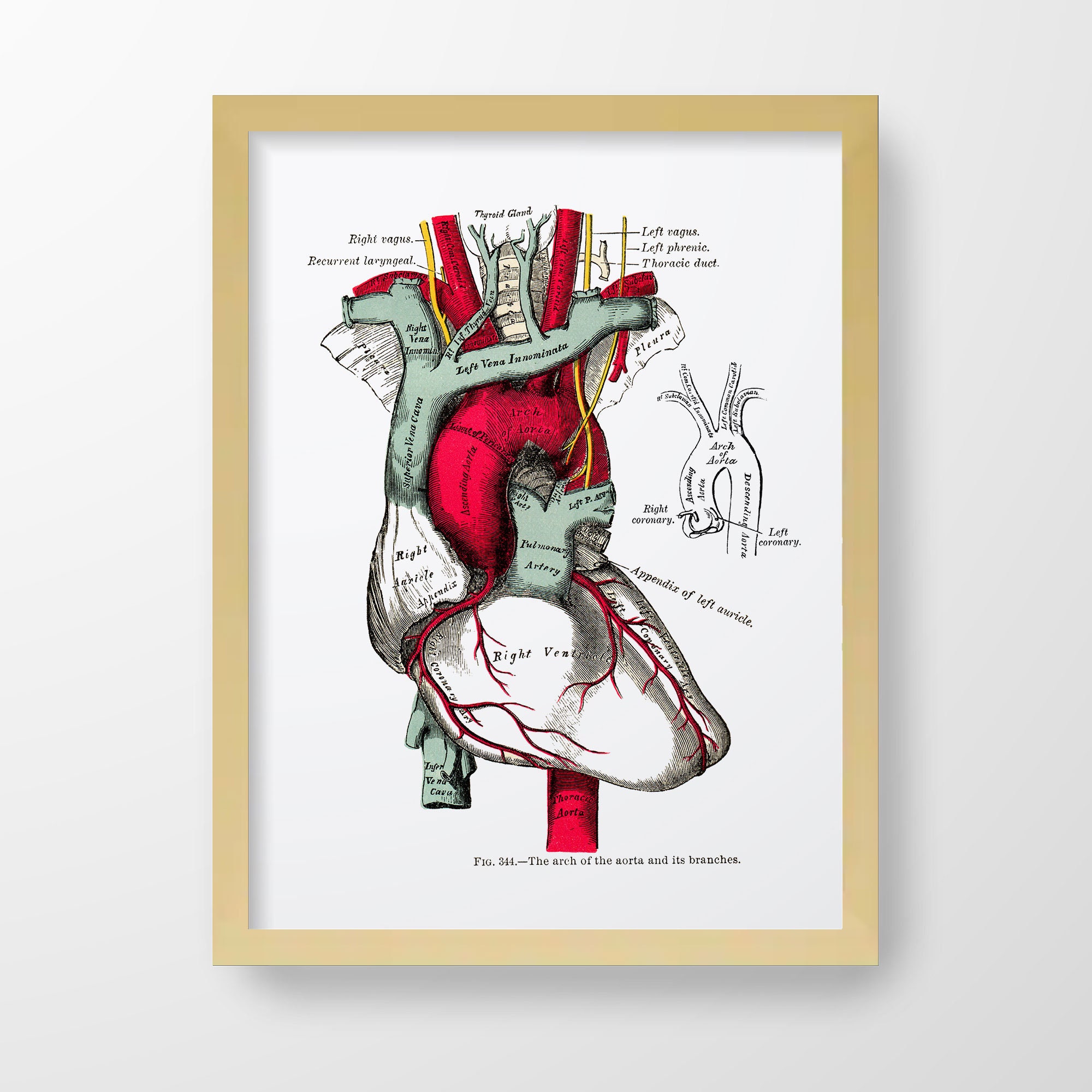The image showcases an artistically rendered medical illustration of a human heart, prominently centered and spanning vertically from the top to the bottom of the frame. The heart is depicted in various hues, including light grayish green, red, yellow, white, black, and grays. It is encased in a light-colored wooden frame, contrasting with the surrounding emptiness of the white background. 

Detailed annotations accompany the illustration, with text labels including "left thyroid duct," "right regis," and other terms that are too small and blurry to decipher clearly. Additional labels mentioned in the text are "figure 344, the arch of the aorta and its branches," "recurrent laryngeal," "right regus," "thyroid gland," "left vagus," "right vagus," "left phrenic," "thoracic duct," "right vena innominata," "left vena innominata," "pulmonary artery," "appendix of left oracle," "right ventricle," "flora," "arch of aorta," "left coronary," and "right coronary." The style of the illustration is distinctly artistic, blending medical accuracy with creative visual presentation.